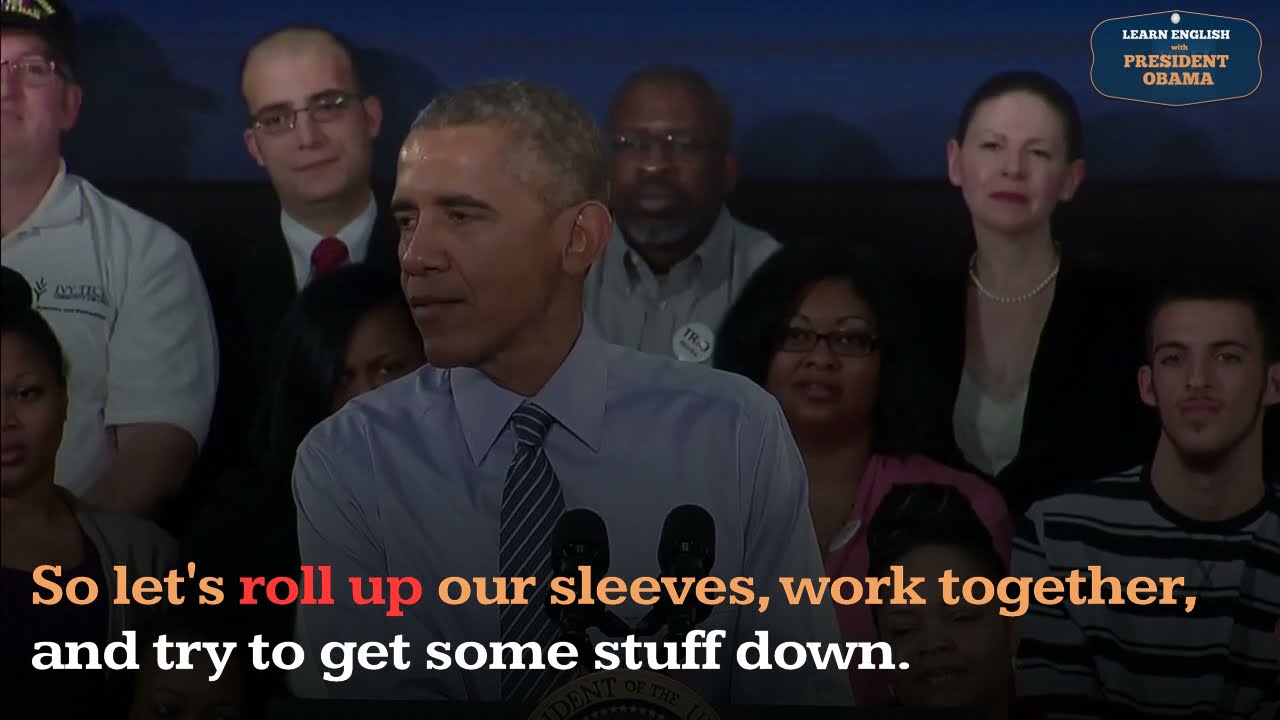The image captures Barack Obama delivering a speech, likely from a campaign or press conference, with a distinctive instructional purpose. At the top right of the image, there is a logo framed in blue with gold trim, reading "Learn English with President Obama." Obama stands at a podium adorned with the presidential seal and dual black microphones, his head turned slightly to the left as if listening for a question. He is dressed in a blue dress shirt and a striped tie, exuding a composed presence.

The background reveals a dimly lit room with an attentive crowd, their faces barely discernible, intently focused on Obama. In the foreground, bold yellow subtitles overlay the image, featuring the highlighted phrase, "So let's roll up our sleeves, work together, and try to get some stuff done." Specific words like "roll up" are emphasized in red, indicating that this is an educational video using Obama's speeches to aid in learning English. The logo and instructional text suggest that viewers can read along and practice their language skills by following the dialogue presented at the bottom of the screen. 

This detailed composition underscores the dual nature of the image: a significant political moment repurposed as a pedagogical tool for English language learners.